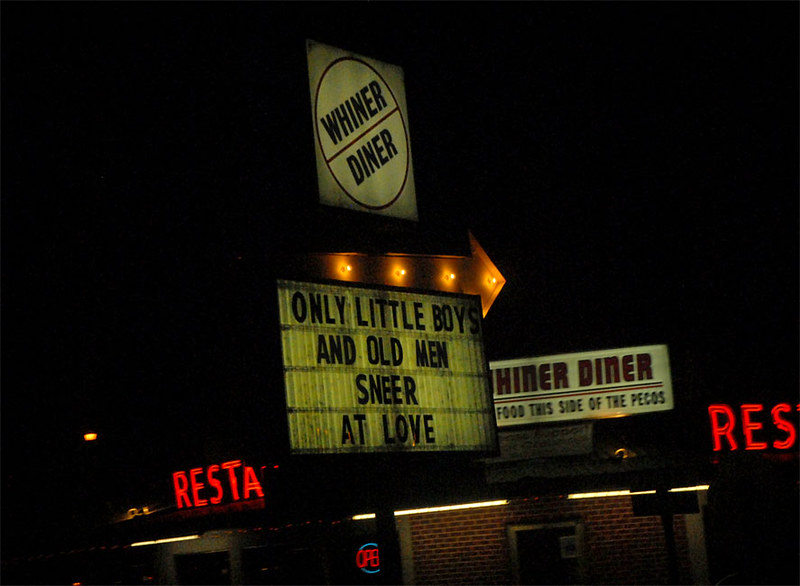In this horizontally-oriented rectangular photograph captured during the dark of night, the viewer's eye is immediately drawn to the illuminated signage set against a black sky. At the top of the image, a square sign facing east prominently displays the words "Weiner Diner" in all capital letters, encased within a rounded inner border. Below this sign, a bright orange arrow also pointing east directs attention to a yellow sign featuring old-fashioned black removable letters that spell out, "Only little boys and old men sneer at love."

To the right of these signs, the Weiner Diner's name is reiterated, juxtaposed with the facade of the building below. The structure is composed of red brick and is topped by a series of red signs that line its upper perimeter, each emblazoned with the word "Restaurant." The scene conveys a nostalgic, almost timeless quality, highlighted by the warm glow of the signage piercing through the night.